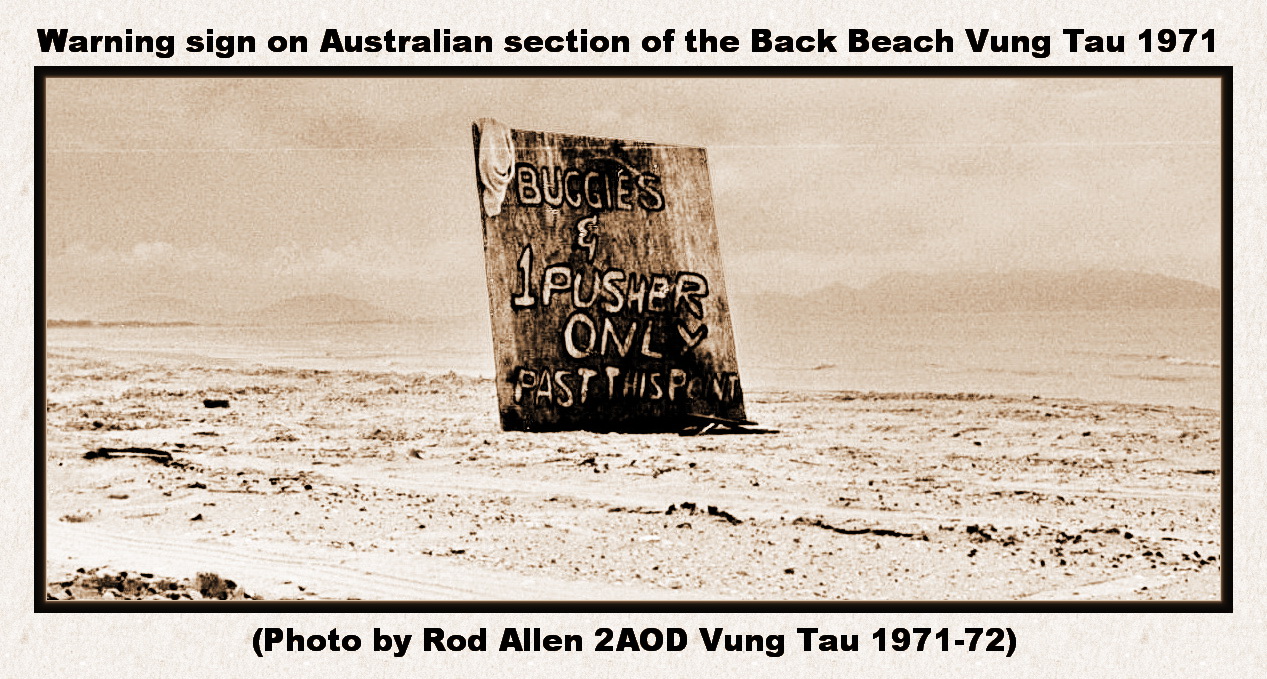This black and white photograph, aged to a sepia tone, captures a hazy scene at the Australian section of the Back Beach in Vung Tau, 1971. Framed by a thin black border, the image shows a beach with sand, ocean waves, and a distant mountain range under a cloudy sky. At the center stands a large, weathered wooden sign with an oddly draped piece of clothing hanging from its left corner. The sign bears a handwritten message in white letters outlined in black, reading: "Buggies and one pusher only past this point." Above the sign, the photograph features a caption that reads: "Warning sign on Australian section of the Back Beach, Vung Tau, 1971." Below, in parentheses, it notes: "Photo by Rod Allen, 2AOD Vung Tau, 1971-72.” The scene evokes a sense of historic caution amidst a serene, yet desolate, landscape.